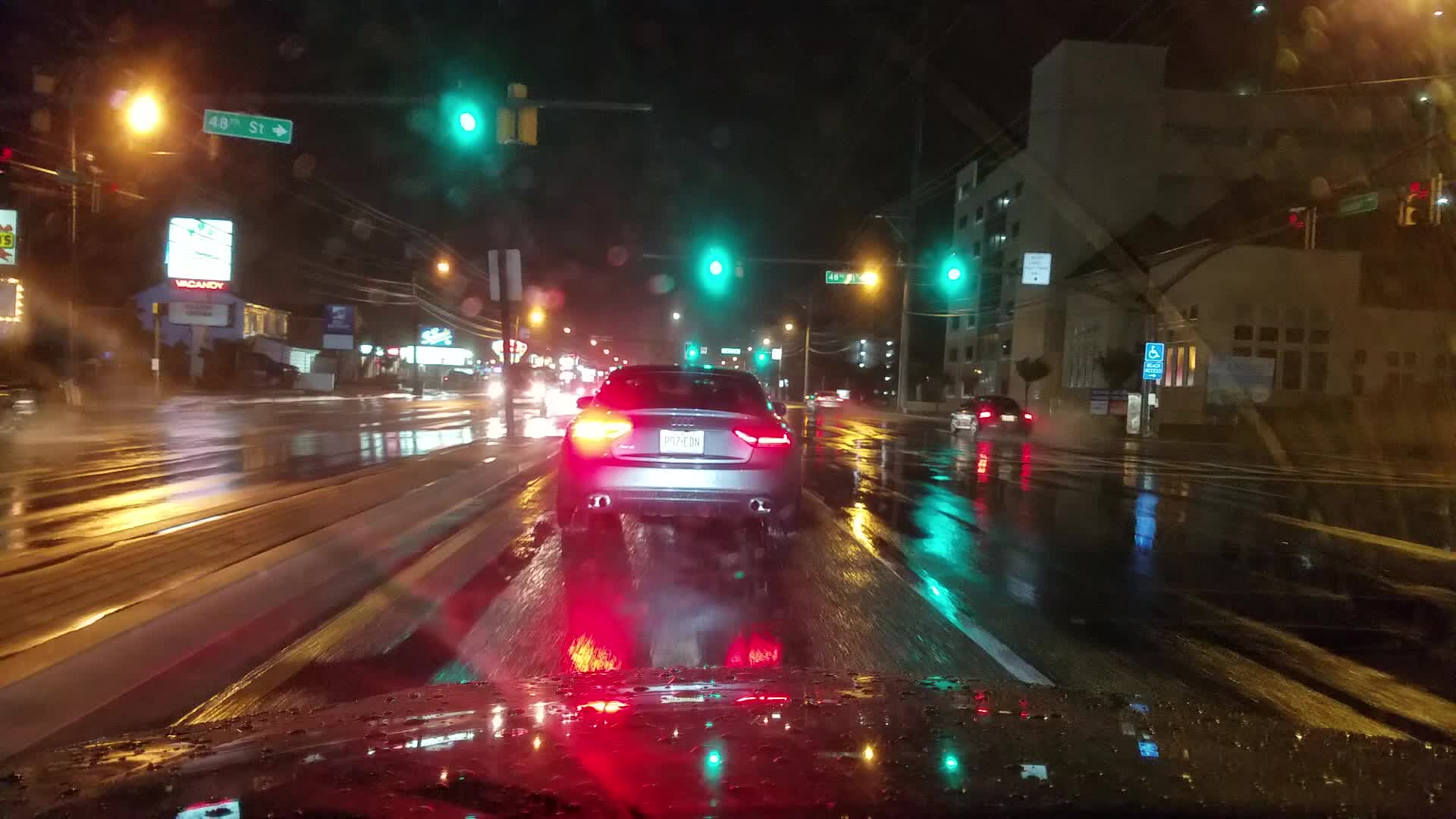In this nighttime photograph, taken from the front seat of a vehicle, either from the driver's or passenger's perspective, the scene captures a rainy street lined with hotels. Directly ahead, a shiny blue car with one functioning brake light and a white license plate waits at a green traffic light. To the right of the blue car, a vehicle with lit headlights is visible but farther ahead in the distance. Overhead and to the left, green street lights illuminate the damp road. On the right side of the street, a tall building, around five stories high, stands prominently with its white or gray exterior. On the left side, a white sign brightly advertises "vacancy," though the text below this is unreadable. The wet pavement glistens under the streetlights, encapsulating the muted hustle of a commercial area filled with hotels.